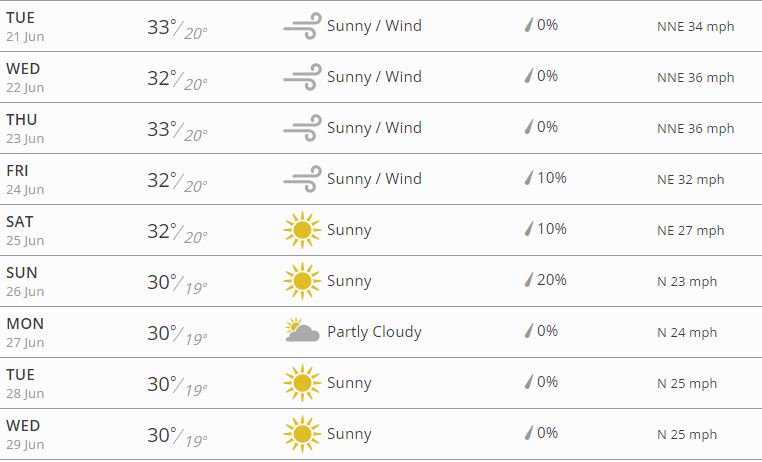The image presents a detailed weather forecast for the week, with an arrangement of symbols and information for each day.

- **Tuesday, 21 June**: Displaying the abbreviation "TUE" on the left side, followed by the date "21 JUN" beneath it. The temperature reads as 33°C in bold black, followed by a slash and a lighter black "20°C". Two long lines curve around at the end, representing wind. A "sunny-wind" icon appears beside a grey raindrop symbol indicating 0% precipitation. The wind speed is noted as North-Northeast (NNE) at 34 mph.
  
- **Wednesday, 22 June**: Shows similar details with a high of 32°C and a low of 20°C. It indicates sunny and windy conditions with 0% precipitation.

- **Thursday, 23 June**: Forecast is almost identical to Wednesday, with temperatures at 33°C and 20°C, sunny-wind conditions, and 0% precipitation.

- **Friday, 24 June**: The temperature displays 32°C/20°C with sunny and windy conditions, and a slight increase to 10% precipitation.

- **Saturday, 25 June**: Shows a high of 32°C and a low of 20°C. The sun icon appears alongside "sunny precipitation" and indicates a 10% chance of rain.

- **Sunday, 26 June**: Displays temperatures at 30°C/19°C, sunny conditions, and a 20% chance of rain.

- **Monday, 27 June**: Indicates temperatures at 30°C/19°C with partly cloudy conditions (represented by a gray cloud in front of the sun), and 0% precipitation.

- **Tuesday, 28 June**: Shows a high of 30°C and a low of 19°C, with sunny conditions and 0% precipitation.

- **Wednesday, 29 June**: Similar to Tuesday, forecasts a high of 30°C and a low of 19°C, sunny conditions, and 0% precipitation.